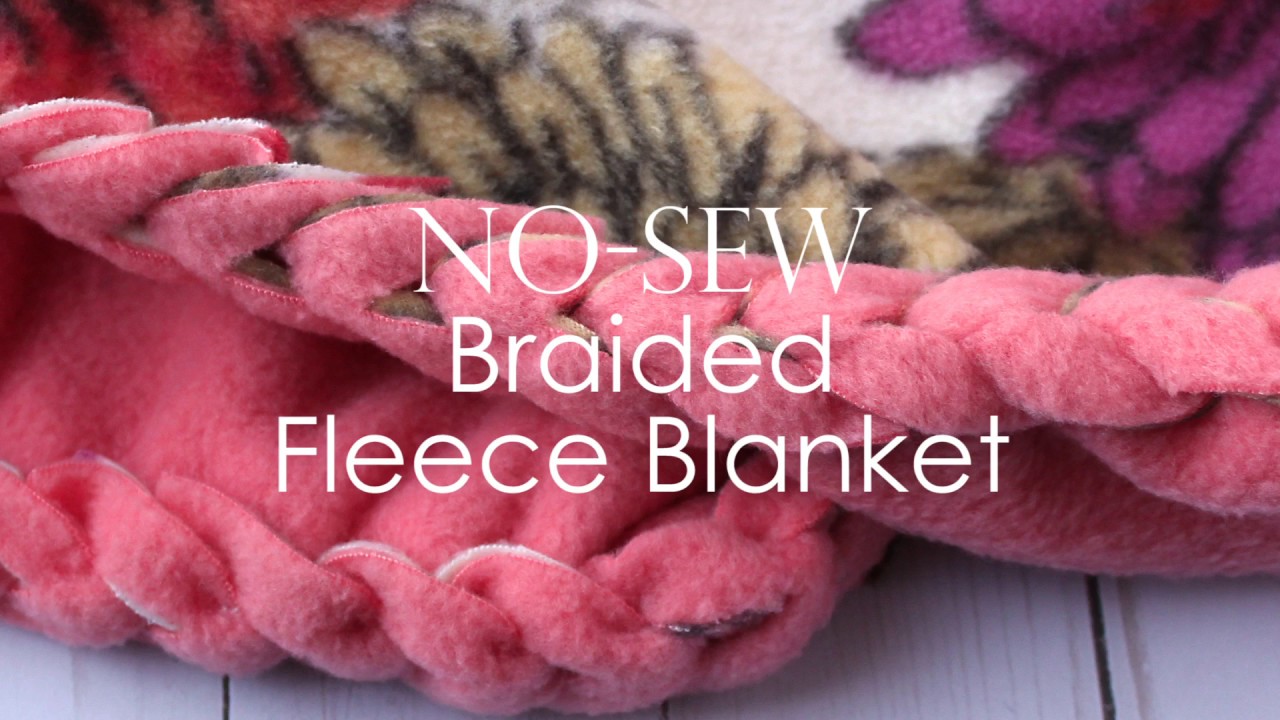The image features a close-up of a fluffy, no-sew braided fleece blanket that appears to be advertised on a blog or in a magazine. The blanket showcases a vibrant palette of pink, purple, and white, with intricate designs including brown plant matter and purple flower petals. It is folded over itself, revealing both the braided pink sections and the detailed floral patterns. Set against a white surface, possibly a table, the blanket exudes softness and warmth. Superimposed over the image in clear, white text are the words "NO-SEW BRAIDED FLEECE BLANKET," emphasizing the DIY nature of the project. The detailed photograph highlights the blanket's cozy texture and appealing design.